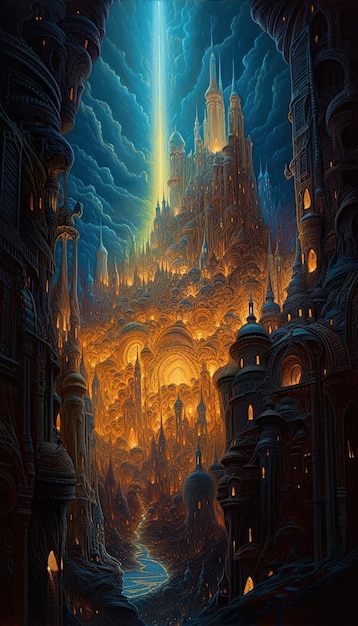This image displays a highly detailed, Van Gogh-esque painting of an ethereal castle, deeply reminiscent of the color palette and whimsical illumination found in "Starry Night." Dominating the scene, a grand, ominous castle with multiple pointy roofs and charming architectural work—reminiscent of Turkish or Islamic styles—perches atop an illuminated mountain. White and blue hues define the castle's peaks, while warm, fire-lit buildings cluster below, casting an orange glow that suggests bustling activity. In the foreground, a serene stream winds its way towards the enigmatic castle. A dramatic light beam splits the heavily clouded sky, directing a severing light towards the heavens and enhancing the painting's mystical ambiance. The intricate play of light and architecture gives the impression that the entire scene is floating, suspended in an otherworldly realm.